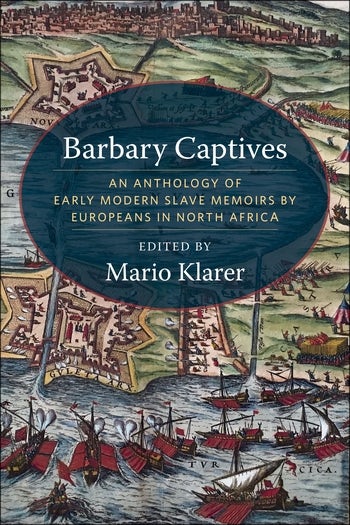The image features the cover of a book titled "Barbary Captives: An Anthology of Early Modern Slave Memoirs by Europeans in North Africa," edited by Mario Klerer. The title and editor information are displayed in an oval section with a blue background, outlined by a thin red line. The background illustration depicts an aerial view of a maritime scene with approximately 12 reddish-brown boats sailing on a blue ocean towards a green land area. The land is marked with brown patches, likely indicating buildings and houses, surrounded by lush green grass. The scene also includes tiny figures on the boats, appearing to navigate towards the shore.